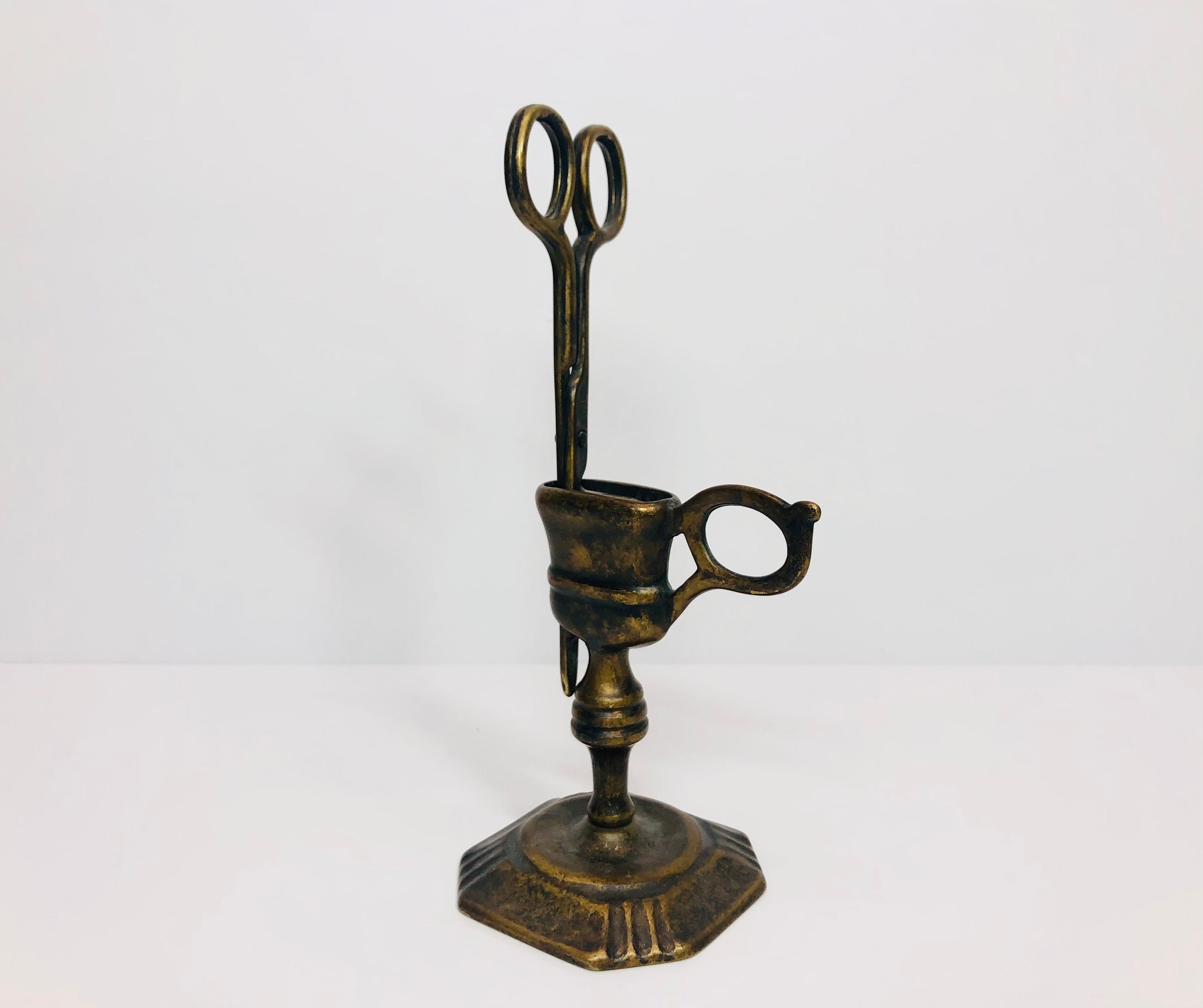This photograph features a meticulously crafted metallic sculpture, giving off an antique and rustic charm with a burnished brass appearance. The piece is displayed against a solid white background and sits on a matching white surface, drawing all attention to its intricate details. It stands on a golden-brown, square base with rounded corners. Rising from this base is a pedestal adorned with concentric rings, culminating in a cup-like structure at the top. Protruding to the right of the cup is a circular handle, reminiscent of a pair of scissors. Inside the cup rests a pair of thick, golden-brown scissors, positioned upright as if ready for use. The composition and focus of the image suggest it could belong to a museum catalog or be used for sales purposes, emphasizing the artifact's form and craftsmanship.